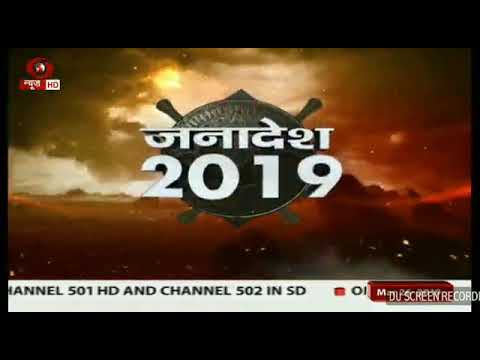The image appears to be a digitally created or screenshot scene, featuring an atmospheric sky as the backdrop. Dominated by rich, vibrant colors, the sky showcases a mix of dark olive green and red clouds, suggesting a dramatic setting, possibly near sunset or during an intense event. The bottom part of the image hints at a dusty red and yellow landscape, adding to the overall intensity of the scene. 

In the center of the image is a large logo, with a rounded symbol and a pair of sticks behind it, both shaded in gray. Positioned prominently over the logo is the number "2019" in bold text. The image is framed by black bars at the top and bottom, likely indicating it is a screenshot, possibly from a mobile device or television. Alongside the logo, in the bottom banner, are the words "Channel 501 HD" and "Channel 502 SD" in white text, alongside additional text in a non-English language, which is also visible in the top left corner.

The overall composition and design give the impression of an advertisement or promotional material for an event or movie, rendered in a style that evokes tension or drama through its color choices and atmospheric elements.